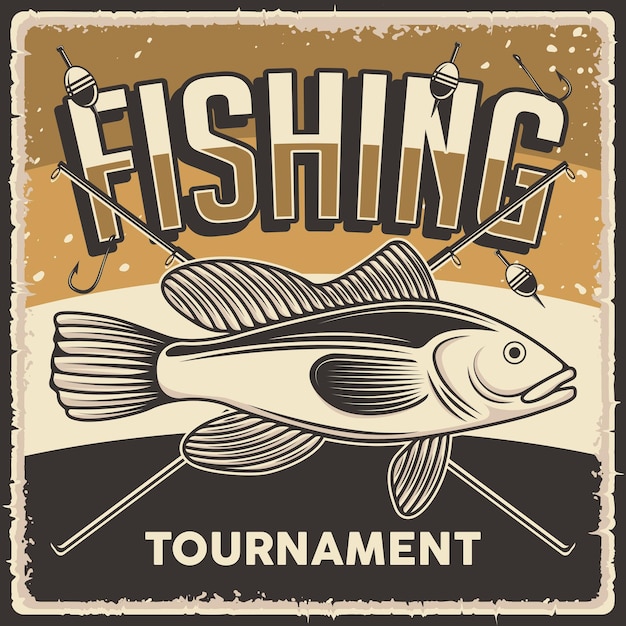This image is a vintage-style graphic of a fishing tournament. The graphic is slightly taller than it is wide and is framed by a frayed cream-colored border with a black edge. The central focus is a large, black and white clipart-style fish, positioned horizontally and facing right, with two crossed fishing rods behind it, forming an X shape. Dangling from these rods are various lures and hooks. The background color scheme primarily features shades of beige, brown, and black. At the top of the graphic, the word "FISHING" is prominently displayed in large capital letters, with a horizontal gradient transitioning from light beige at the top of the letters to medium brown at the bottom. Below the fish, the word "TOURNAMENT" is written in bold, capital white letters set against a solid black section. The overall design and texture give it a nuanced, worn, and vintage appearance, effectively highlighting the event details.